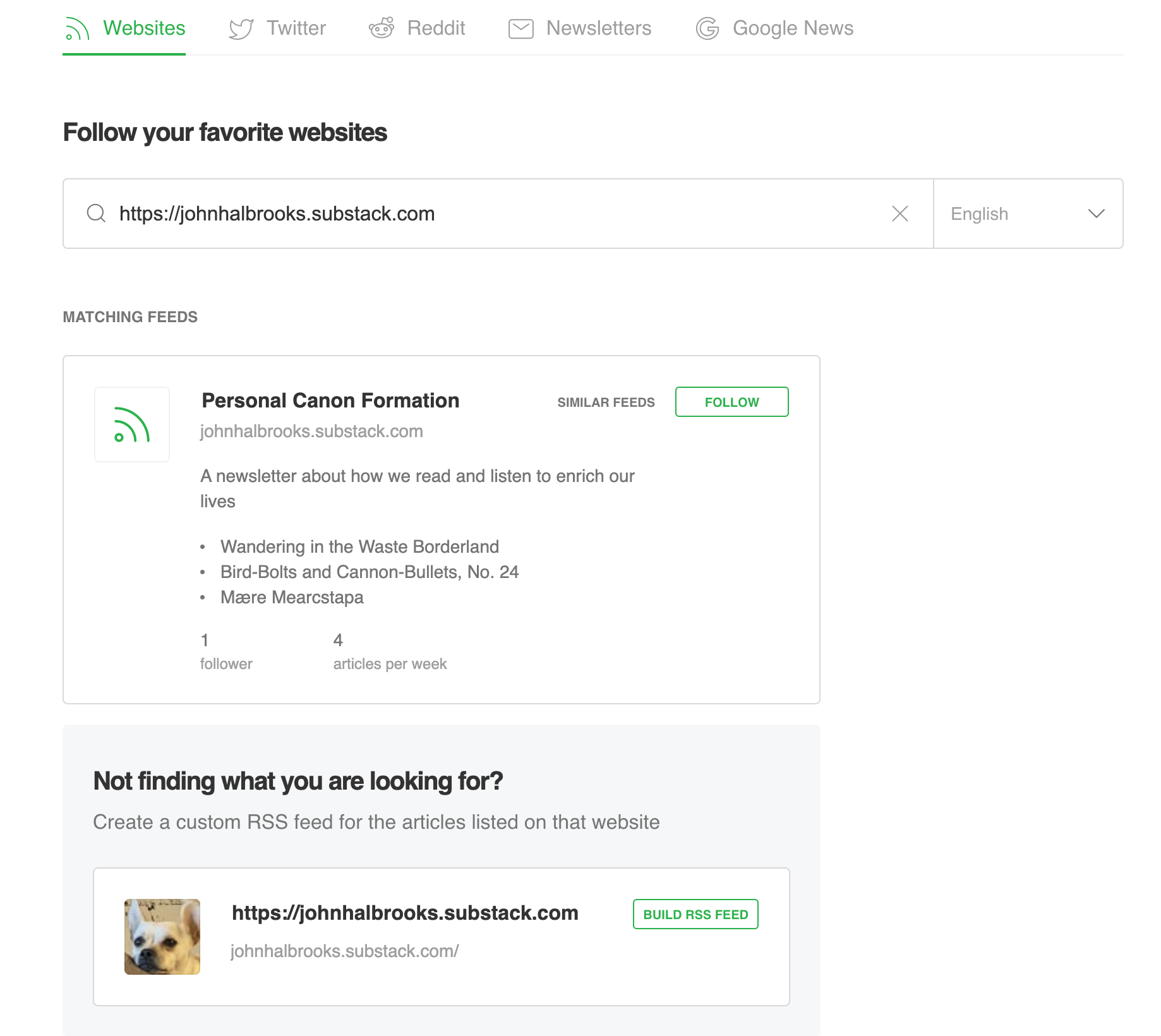The image showcases a computer screen displaying a website tool that allows users to follow their favorite websites. The screen predominantly features a white background. At the top of the interface, there are five clickable options: "Websites" highlighted in green with an accompanying website icon to its left, and "Twitter," "Reddit," "Newsletters," and "Google News" in gray with corresponding logos.

Centrally positioned is a prominent, dark black heading that reads, "Follow your favorite websites." Directly below is a search field bordered by a thin gray line, containing a small magnifying glass icon and pre-filled with the URL "https://johnhallbrooks.substack.com". At the far right of this field, there's a small "x" button, and to its right is a drop-down menu indicated by a downward-facing caret symbol, with the word "English" displayed.

Further down the screen, there's a section titled "Matching Feeds." Within this section is a rectangular panel outlined in thin gray lines. At the panel's top, in dark letters, it reads "Personal Canon Formation" followed by the cited website "johnhallbrooks.substack.com". To the left of these words is a green symbol matching the one seen next to "Websites". To the right, in smaller text, it says "Similar Feeds," accompanied by a green-outlined button labeled "Follow."

Descriptive text below this panel mentions: "A newsletter about how we read and listen to enrich our lives." Three bullet points are listed as follows:
- "Wandering in the Waste Borderland"
- "Bird Bolts and Canon Bullets, No. 24"
- "Mayor Maersk DAPA"

Additionally, it notes "1 follower" and "4 articles per week."

At the bottom, there's a gray rectangular panel with the heading, "Not finding what you're looking for?" followed by a smaller gray subheading, "Create a custom RSS feed for the articles listed on that website." Inside this gray panel, there's a white rectangular box featuring an image of a dog on the left and the website URL "https://johnhallbrooks.substack.com" next to it. To the right of the URL is a green-outlined button with the text "Build RSS Feed."